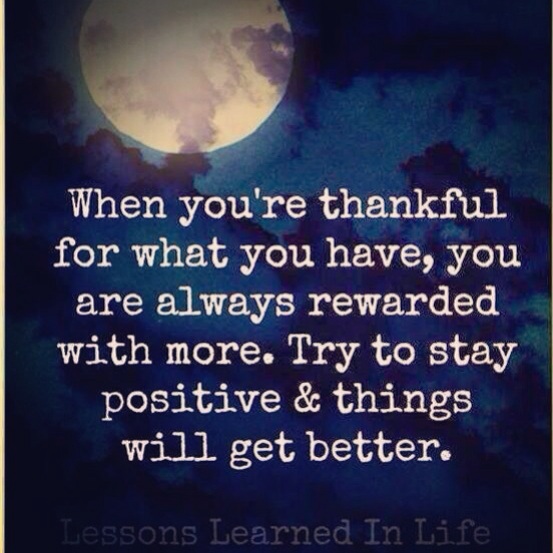The image is an artistic graphic featuring a dark, night sky. Dominating the upper left corner is a large, white full moon that illuminates the scene. Scattered dark blue and black clouds are visible, contrasting against the moon's bright shine. In the center of the graphic, there's a poignant quote printed in a white font: "When you are thankful for what you have, you are always rewarded with more. Try to stay positive and things will get better." At the bottom of the image, in a dimmer gray font that blends into the almost entirely black lower section, the text reads: "Lessons learned in life." The moonlight serves as the primary light source, highlighting the elements of this serene nighttime scene.